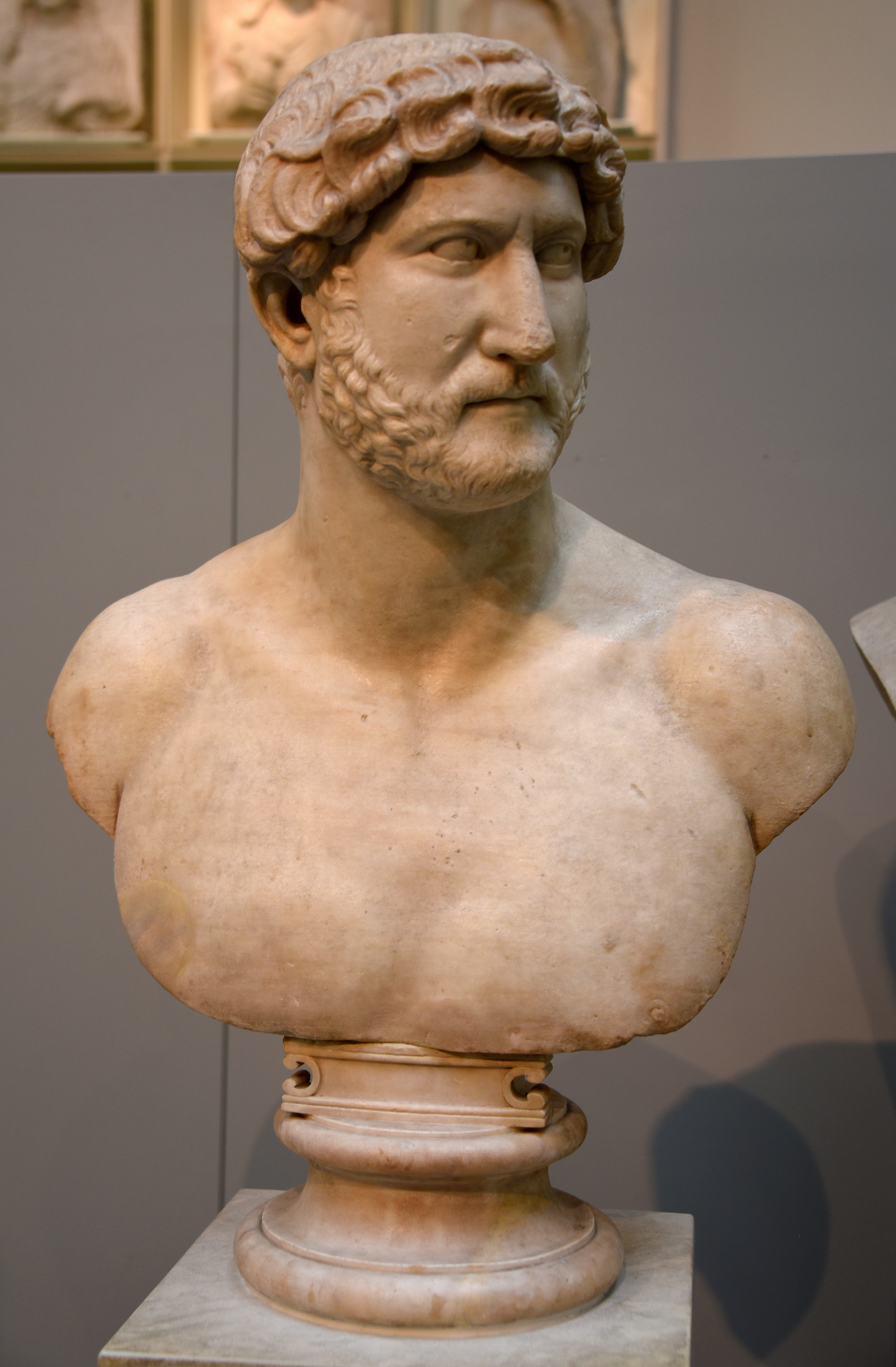The photograph captures a detailed statue bust of a historical figure, likely a Greek man, set against a predominantly dark gray museum backdrop with faint lighter gray areas at the top. This life-like bust features the man's large nose, short curly hair that is somewhat feathered or wavy, and a curly beard and mustache. His head is angled slightly to the left, exuding a noble demeanor. The statue, made from a light tan or cream-colored material with a few chips and dings, includes broad shoulders and part of the upper chest, with his left nipple visible. The bust is mounted on a white pedestal, though only the top of it is visible in the image. Behind the statue, there appears to be a plaque or temporary wall, adorned with stone-carved artwork that is slightly blurry, hinting at the museum setting. No text or identification is provided, adding an air of mystery to the depicted figure.